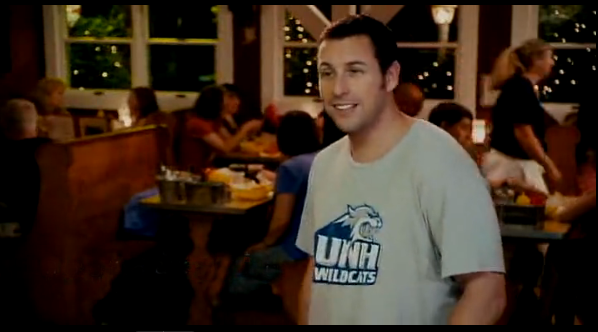The image depicts actor Adam Sandler, positioned on the right side, with short brown hair, smiling broadly with his mouth open, revealing his top row of teeth. He is wearing a gray sweatshirt emblazoned with a UNH Wildcats logo, featuring an illustrated wildcat. The setting appears to be a bustling restaurant or diner, identifiable by the numerous tables and booths behind Sandler, populated with people dining and enjoying meals. The background is characterized by large windows through which the night sky is visible, along with stringed lights adorning trees outside, suggesting a festive, possibly holiday atmosphere. A waitress can be seen in the background to the right, tending to the busy scene, which is well-lit and conveys a lively, sociable ambiance. The overall impression is reminiscent of a still from a movie, capturing a candid moment amid a vibrant dining environment.